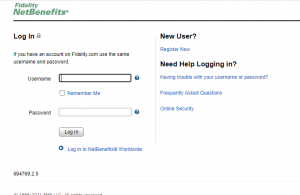This image is a low-resolution screenshot of a Fidelity NetBenefits page, presented in a horizontal landscape orientation. Despite the grainy quality, it is possible to decipher several key elements. 

In the top left corner, "Fidelity NetBenefits" is displayed in green italicized text. Beneath this heading, a black horizontal line separates it from the login area. Here, users are instructed to use their Fidelity.com username and password. There are input fields provided for the username and password, accompanied by a "Remind Me" option with a checkbox. Below the password field, a gray button labeled "Log In" invites users to access their accounts, though the text following "Log In to..." is illegible due to the blurriness. A number is also present in the bottom left corner, but it is too unclear to read.

On the right side of the image, there is black text that says "New User" above a blue link that reads "Register Now." Further down, black text asks "Need help logging in?" and addresses common issues with usernames or passwords. The section concludes with links to "Frequently Asked Questions" and "Online Security" at the bottom.